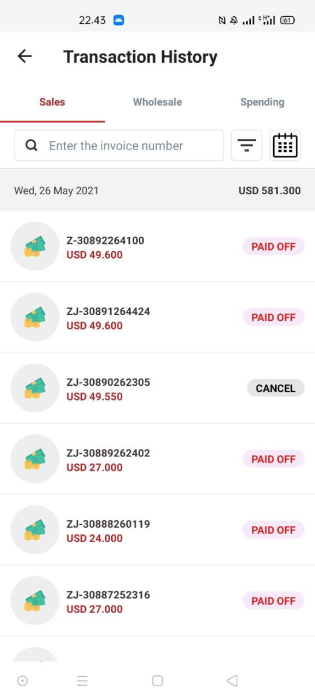This is a screenshot from a cell phone display at 22:43. The status bar at the top indicates the current time, shows a weather icon, has NFC enabled, and an active alarm. It also displays the network status and battery life. The primary app visible is a transaction history page, seemingly for a store management system. The app is on the "Sales" tab, next to "Wholesale" and "Spending" tabs. Below these tabs is a search bar labeled "Enter the invoice number," accompanied by filter and calendar icons for refining the view of transactions. The detailed transaction list starts with an entry dated Wednesday, 26th May 2021, showing an amount of USD 581.300, followed by several other transactions. Each entry includes specific details such as date and transaction amounts, although the format displaying several decimal places is unusual.